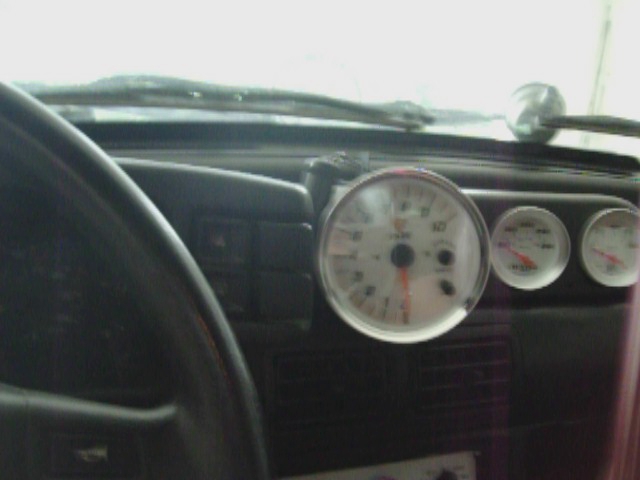In this somewhat blurry photograph, a modern vehicle's dashboard is depicted with a left-side steering wheel. Dominating the center of the dashboard is a large, round gauge, possibly a speedometer or tachometer. Flanking this central dial are two smaller round gauges, though their details remain indistinct due to the blurriness. Interestingly, these gauges appear to be retrofitted in a space where the vehicle’s radio might typically be located, suggesting perhaps that the original speedometer or tachometer is non-functional and necessitating this modified setup for essential display readings.